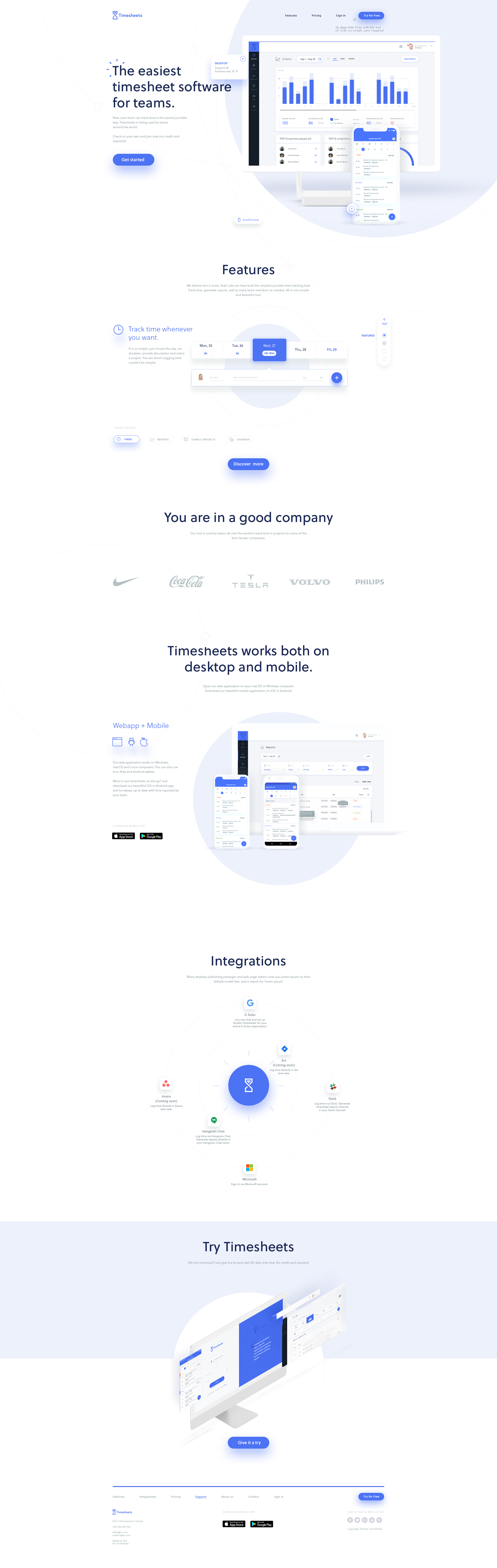This image appears to be a screenshot of a webpage, likely from a computer screen, promoting a timesheet software for Teams. At the very top left corner, there's a snippet of text mentioning timesheets. The main part of the image features a blue area with bar graphs, likely showcasing data visualization capabilities of the software. Below the graph section, there's a section detailing the software's features, followed by a statement that says "You are in good company," suggesting user testimonials or endorsements. Towards the bottom middle, there's a section labeled "Integrations," depicted with a blue oval shape that branches out into six sections, three at the top and three at the bottom, possibly listing compatible applications or platforms. Finally, at the bottom of the image, there's a light blue rectangle with a call-to-action button that says "Try Timesheets." On the right side of the image, there's a graphic of a computer monitor displaying both blue and white screens, reinforcing that this is an advertisement encouraging users to try the timesheet software.